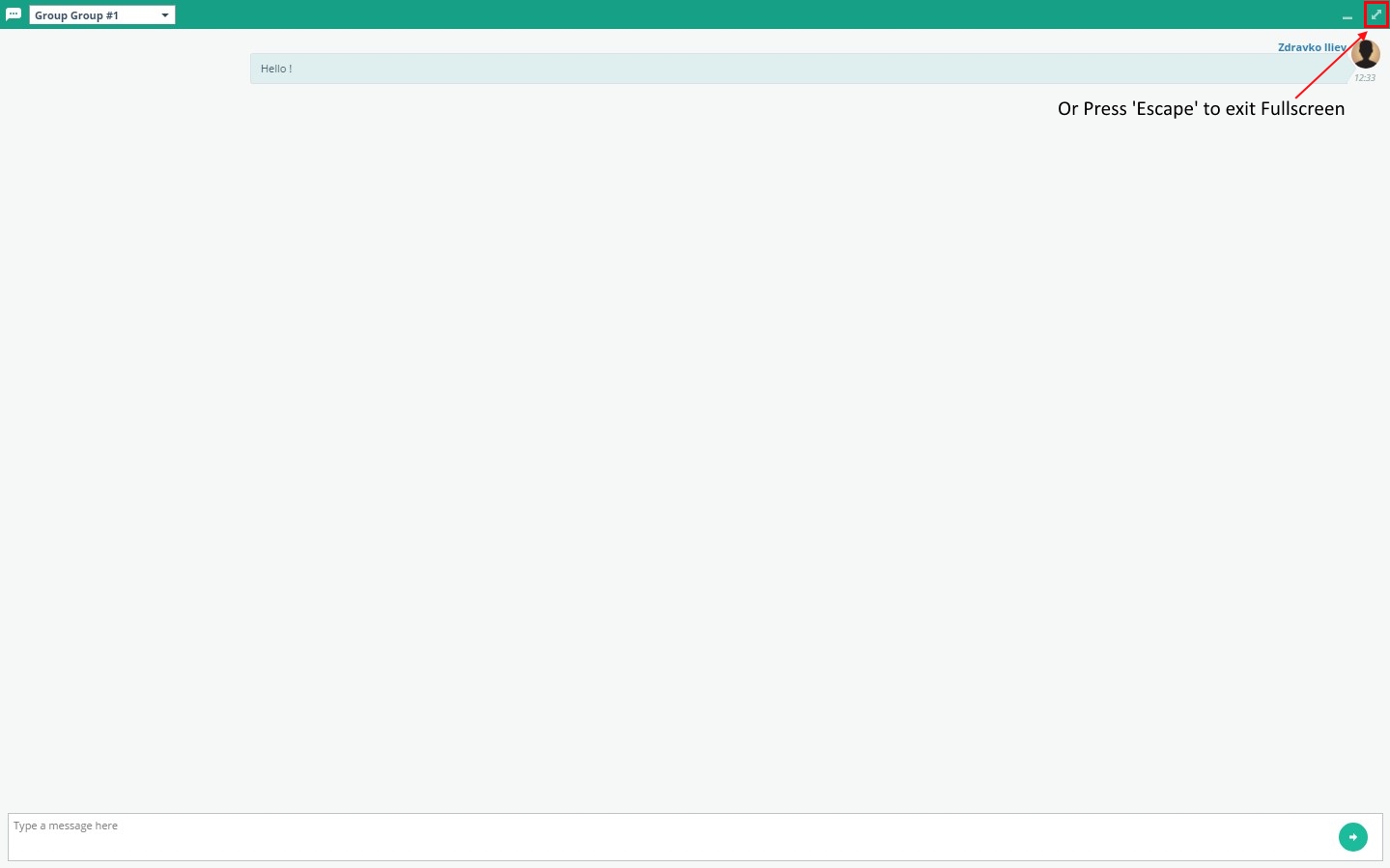This image is a computer application screenshot that prominently features a teal-blue header at the top. On the left side of the header, there is a message box icon, and to its right, a drop-down menu currently displaying "Group Group 1." In the top right corner of this header, there are minimize and maximize icons, with the maximize icon highlighted in a red square. A red arrow points to this icon from the bottom left, accompanied by black text that reads, "or press Escape to exit fullscreen."

Below the header, the main body of the application has a light grey background. There is a wide rectangular chatbox in the middle with "Hello!" typed into it. To the right of this chatbox, there is a profile picture in the form of a brown circle containing a black silhouette of a person, labeled "1233." Above the chatbox, the text "Shedravko Iliev" appears in blue with the detailed spelling "Z-D-R-A-V-K-O-I-L-I-E-V" underneath it.

A large area of negative space lies below this chatbox, leading to a message input box at the bottom. This input box is a white rectangle outlined in light grey, with "Type a message here" written in the top left corner. On the right side of this input box, there is a teal circle featuring a white arrow pointing to the right.